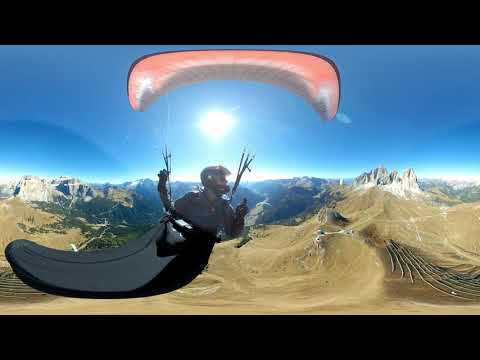The image depicts a man suspended in mid-air by a large, salmon-colored parachute, which he holds onto via two straps. The top half of the image features a light blue sky with a bright white circle representing the sun positioned above him. The parachute stretches across the upper portion, and there is a faint reddish hue with a black outline in the background. The man, wearing a helmet and a long gray shirt, is visible from the chest up and appears to be nestled inside a large, banana-shaped, gray and black sleeping bag-like object. This object runs horizontally across the lower part of the image. Below this, the scenery unfolds into a vast, desert-like landscape with brown and tan hues, interspersed with peaks of stone mountains. Further in the distance, the terrain transitions from barren to forested green, culminating in snow-covered mountaintops under the deep blue sky.